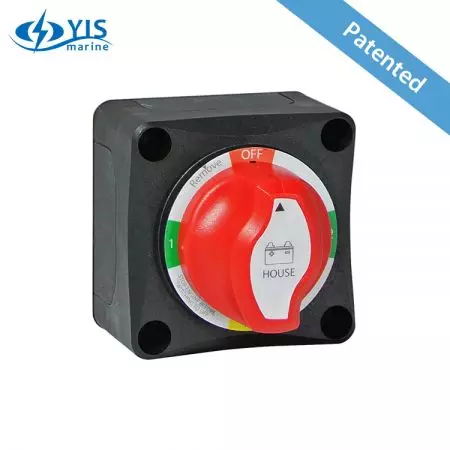This is a full-color, professionally photographed sales ad for a marine battery switch by YIS Marine. The primary focus is a compact black box with a prominent red dial at its center. The dial features a white label adorned with a black arrow and a diagrammatic representation of a battery, indicating the "house" terminal. The switch is set to the 'off' position but offers multiple selectable options including "remove," "1," "2," and "on" as indicated by the various colored sections: red (off), green (1), green (2), and yellow (on). The box has black circles, presumably mounting holes, at each corner. In the upper part of the image, the YIS Marine logo—a blue circle featuring a lightning bolt flanked by crescent moons—appears alongside a blue banner declaring the product as patented. The background is stark white, amplifying the visibility of the switch's details and the YIS Marine branding.